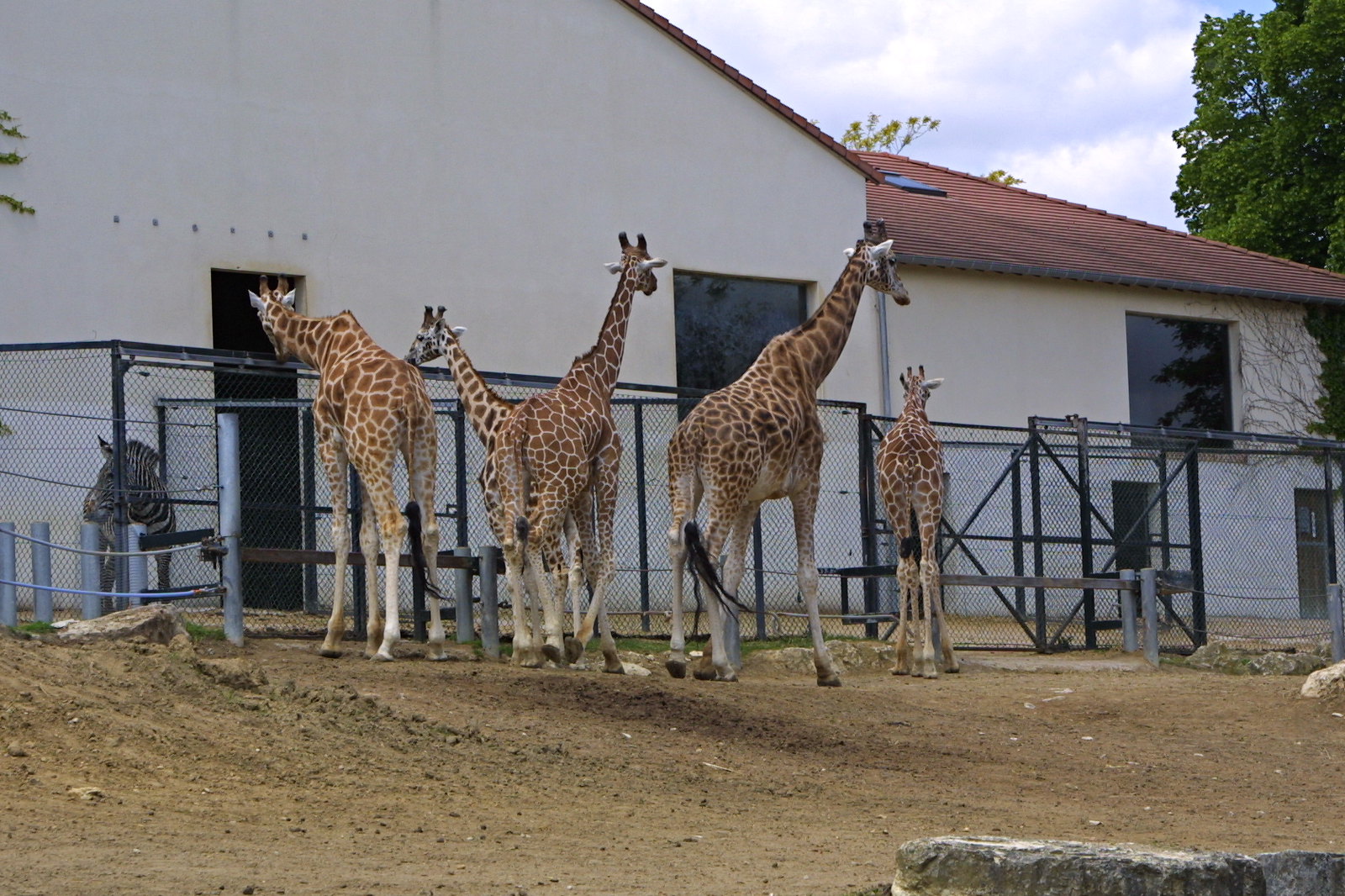In this detailed outdoor photograph taken at a zoo, the central subjects are five giraffes and one zebra situated against a sandy ground populated with pebbles and larger rocks. The giraffes, including two juveniles, display their signature yellow-orange coats with brown patches. They are mostly facing away from the camera, with two on the left leaning over a chain-link fence as if trying to interact with the zebra. The zebra, easily identifiable by its black and white stripes, stands inside an enclosure on the left side of the image.

Dominating the background is a large, tan building with flat walls, crowned by a red Spanish tile roof that pitches from right to left. The building features large square single-pane windows and a tall, open doorway on the left. Adjacent to the building, a chain-link fence with black supports delineates the enclosures and pathways within the zoo. Above, a blue sky filled with cumulus and nimbus clouds stretches across the top of the frame, and the upper right corner reveals the leafy branches of a very tall tree. This richly detailed scene captures a tranquil moment among the zoo animals, highlighting both their beauty and their enclosed surroundings.